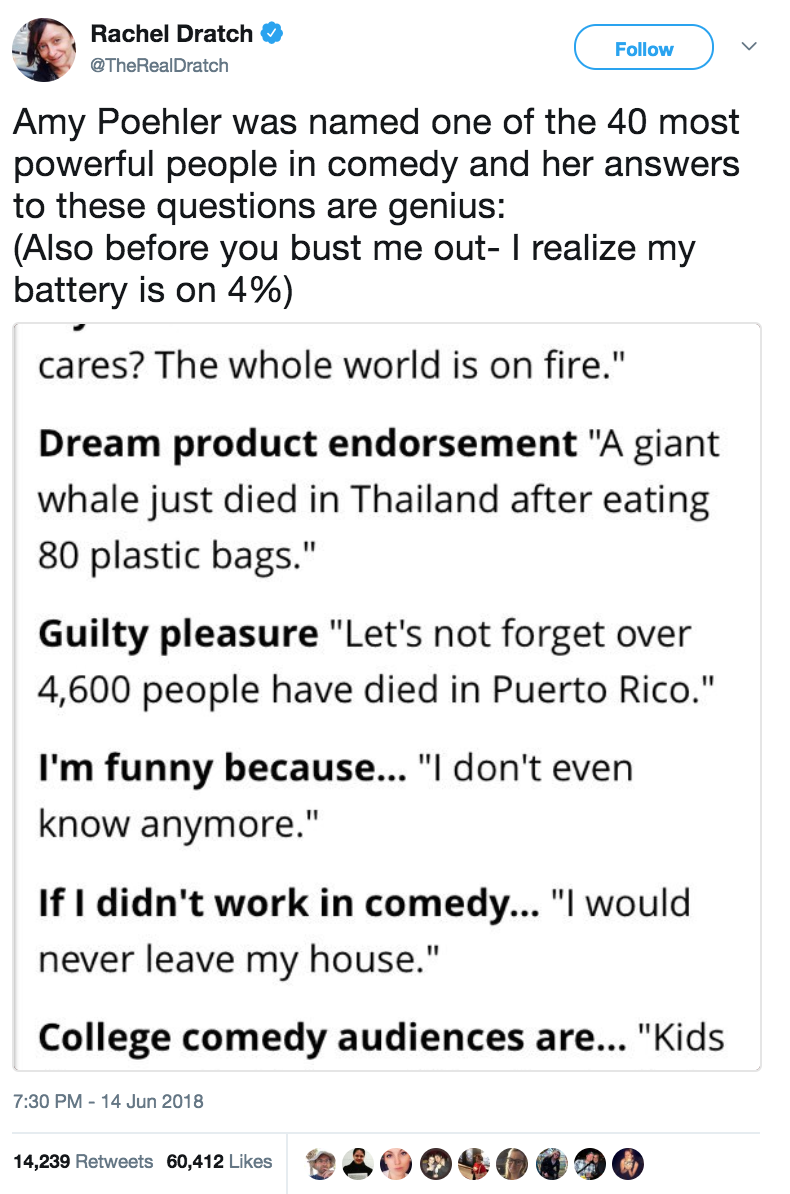This is a detailed screenshot of a post on what is now called X, formerly Twitter, from Rachel Dratch, whose verified handle is @TheRealDratch. The profile picture features Rachel Dratch, and her verification is indicated by a blue checkmark next to her name. The post reads, "Amy Poehler was named one of the 40 most powerful people in comedy, and her answers to these questions are genius. Also, before you bust me out, I realize my battery is on 4%."

The screenshot within Rachel's post displays a set of questions answered by Amy Poehler, with her thoughtful and poignant responses:

1. **Dream product endorsement**: "A giant whale just died in Thailand after eating 80 plastic bags."
2. **Guilty pleasure**: "Let's not forget over 4,600 people have died in Puerto Rico."
3. **I'm funny because**: [The answer is not visible in the provided screenshot.]

Rachel's commentary highlights Amy Poehler's influence and the sharp, socially conscious nature of her responses to the questions.